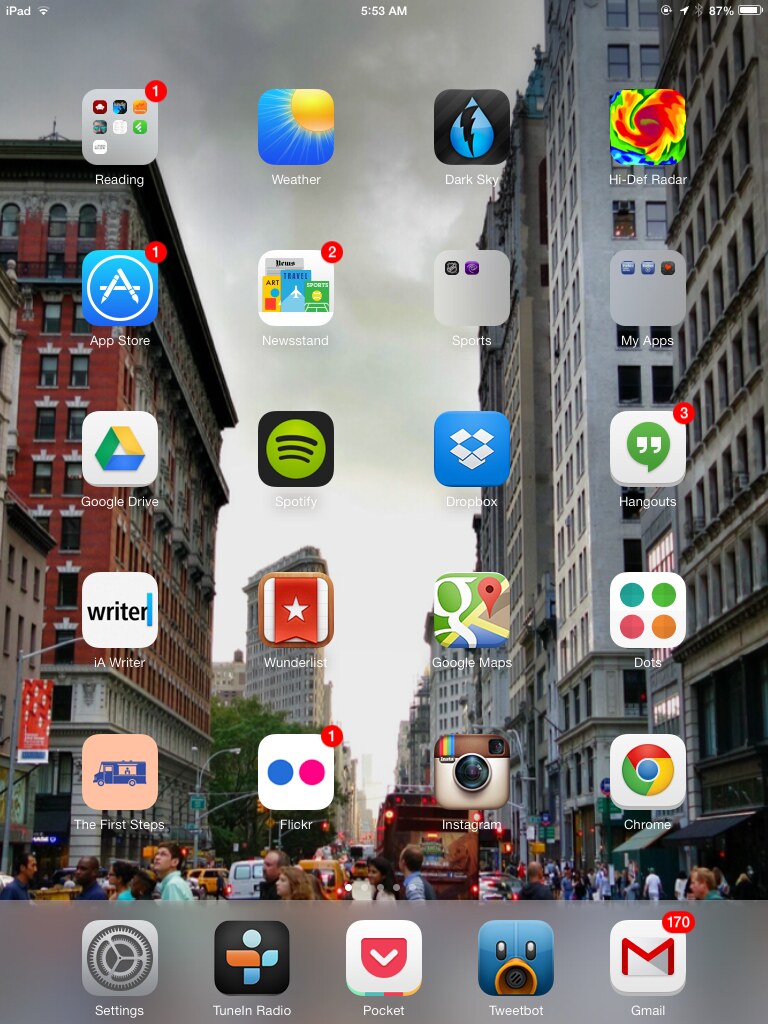This image showcases the cover page of an iPad screen, filled with a variety of app icons. At the bottom, the main icons displayed are Settings, TuneIn Radio, Pocket, TweetBot, and Gmail. Above these, there are 20 additional app icons arranged in neat rows of four. 

The iPad screen has a background depicting a lively street scene in New York City, prominently featuring the Flatiron Building and Square in the background. The foreground reveals a bustling street filled with numerous pedestrians and vehicles, flanked by tall buildings on either side.

Among the icons positioned above the main set at the bottom, notable apps include Chrome, Google Maps, Hangouts, High Def Radar, the Apple App Store, Google Drive, and Dropbox. There are also several gray folders containing smaller icons inside, indicating collections of related apps.